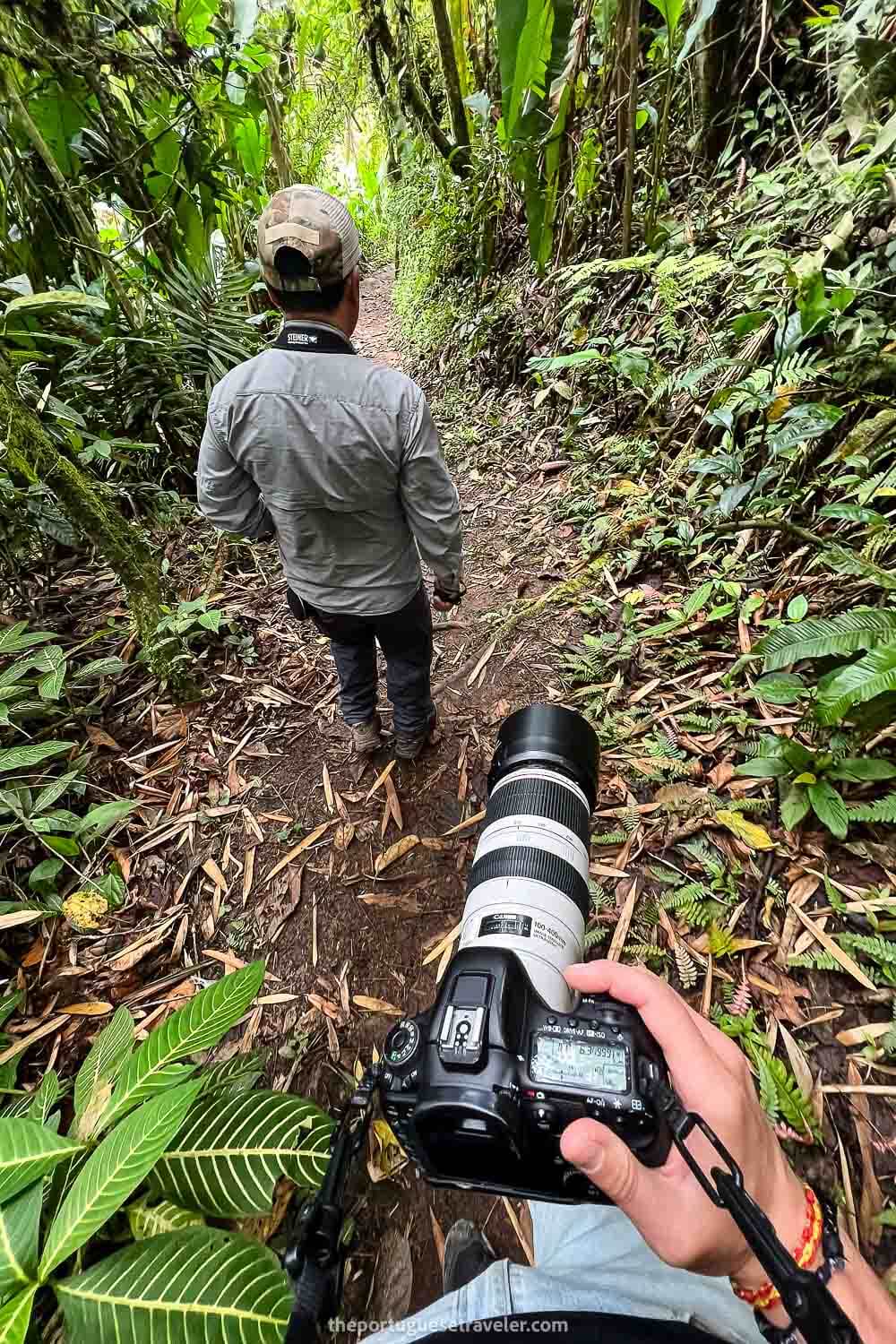In this intricate photograph, two individuals traverse a narrow, dirt-laden path within a verdant, tropical jungle teeming with lush foliage characterized by large, green leaves, some streaked with cream-colored veins. The person in the foreground, partially visible from the waist down, wears blue jeans and holds a professional DSLR camera with a substantial white telephoto lens, hinting at keen interest in photography. His right wrist adorns woven bracelets in red, yellow, and black hues. The man ahead, largely seen from behind, dons a camouflage baseball cap and a long-sleeved gray shirt paired with dark jeans and work boots. A camera strap is evident around his neck, suggesting he, too, might be indulging in photography. The surrounding flora stands tall on both sides of the trail, creating a vivid green canopy that enhances the tropical ambiance. At the bottom of the image, faint white text reads "theportuguesetraveler.com," subtly branding the scene with the photographer's signature.